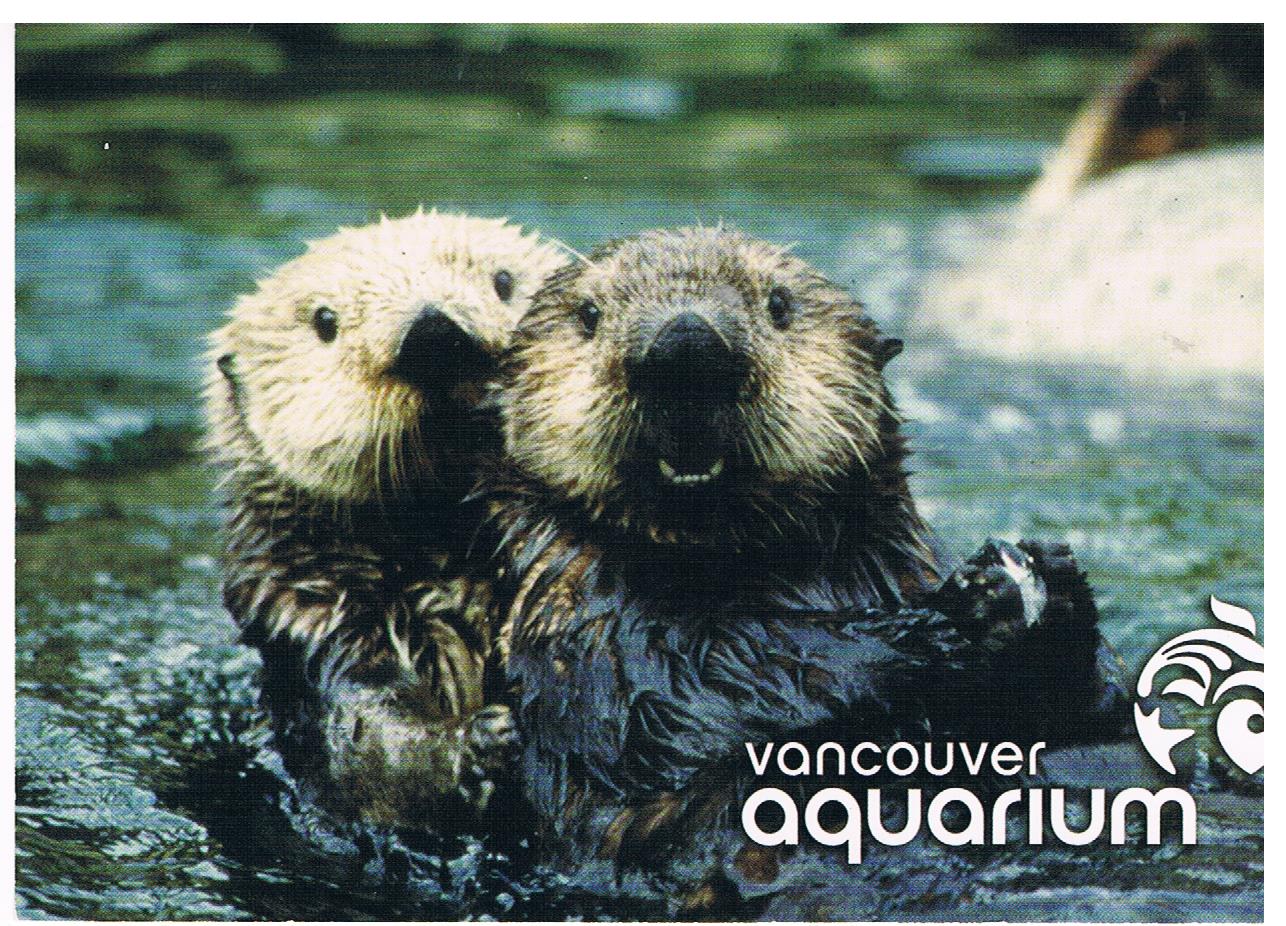In a photograph reminiscent of an old postcard, two wet, brown-furred otters are partially submerged in a churning, light green to blue water. The otters, with lighter brown faces, tiny black beady eyes, and black noses, are warmly embracing each other — the one in the back wrapping its arms around the front one while the front otter holds a small shellfish. Both otters are gazing directly into the camera, seemingly smiling. The water around them is rippling with movement. In the lower right corner of the image, a white logo of a jumping fish with the words "Vancouver Aquarium" is superimposed. In the background, a blurry brownish object is faintly visible.